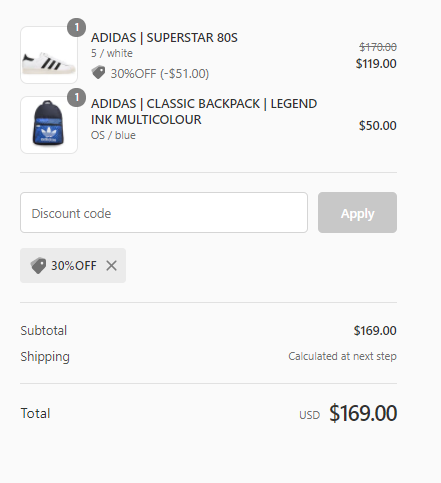**Image Caption:**

The screenshot depicts an online checkout page for Adidas products, displaying two main items and their respective prices. The first item is the Adidas Superstar 880 S5 White Tennis Shoes, identifiable by their white color with classic black stripes. Originally priced at $170, they are now available at a discounted price of $119. The second item is a Classic Backpack in Legend Ink Multicolor OS/Blue, priced at $50.

Above the listed shoes, there's a smaller image of the backpack. The checkout interface includes a field to enter a discount code, currently showing a 30% discount being applied. The subtotal for the items comes to $169, with shipping costs to be calculated in the next step. The total amount displayed is $169.00 USD.

The page is designed with a white background and predominantly black and gray font. The input field for the discount code stands out with a brighter white shade compared to the off-white background of the website.